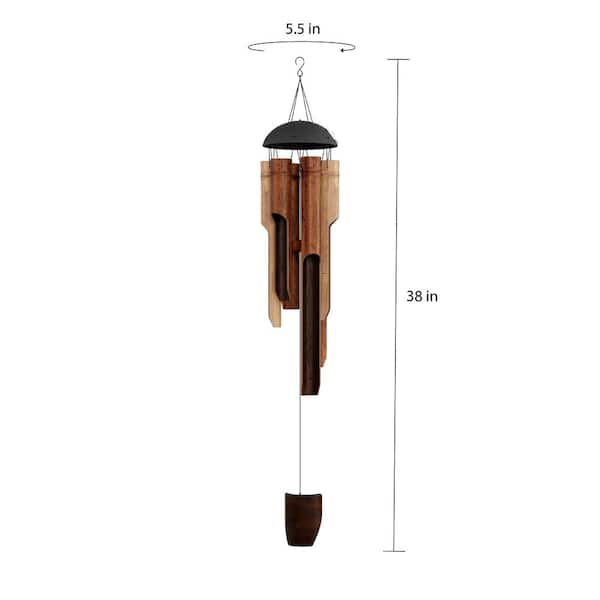The image is a detailed diagram of bamboo wind chimes against a flat white background. Central to the illustration is a series of bamboo chimes in varying lengths, colored brown with black finishes. They hang from a domed top, also black, and are suspended by strings that converge at a small hook meant for hanging. The total height of the wind chimes, measured from the hook to the small bamboo wind catcher at the bottom, is marked as 38 inches with a line on the right side, depicting this dimension. Additionally, an infographic at the top indicates the circumference of the chimes, which is 5.5 inches. The entire image, crafted with a watercolor or illustrative style, provides a clear, concise representation, making it suitable for use on packaging or educational materials.